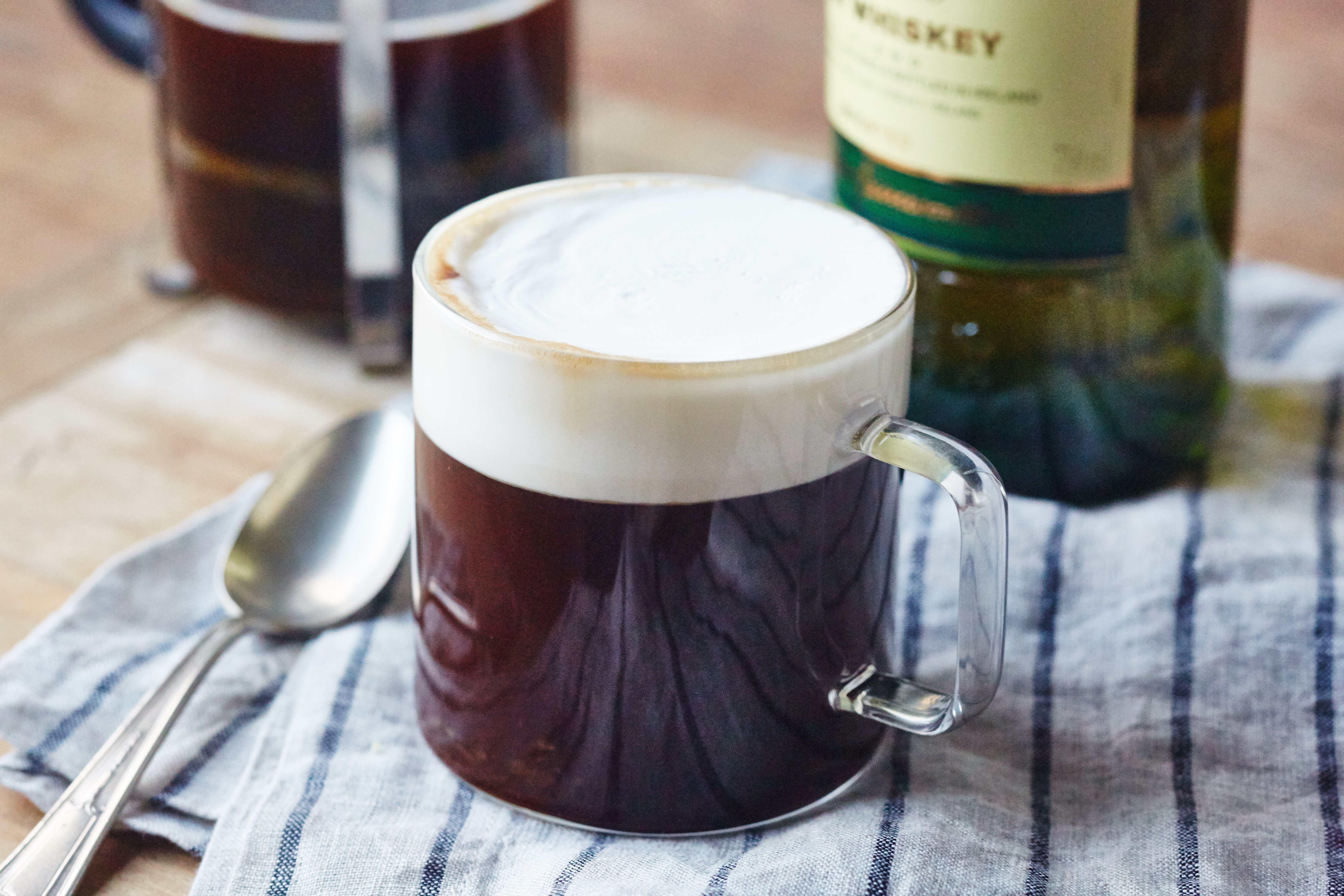The image captures a close-up shot of a see-through glass mug containing a dark brown beverage, which appears to be a combination of coffee and whiskey. The drink has a frothy top that covers around 2 centimeters of the mug. The mug sits on a blue-and-white striped cloth on a wooden table. Adjacent to the mug is a metal spoon, and in the blurred background, there is the lower half of a green bottle labeled "whiskey" and a French press containing black coffee. The clear focus is on the glass mug and its intricate details.